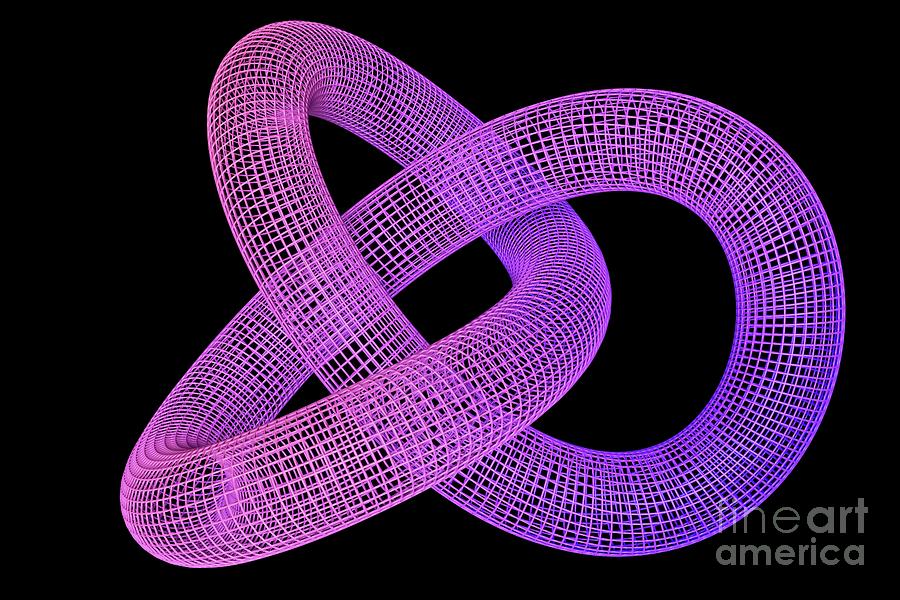This image showcases a 3D-rendered digital artwork featuring a complex, twisted structure that resembles interlocking rings or an infinite coil, made of large, see-through mesh tubes. The tubes start with a soft pink hue and gradually shift into shades of purple and blue as they twist and loop into one another, forming a shape reminiscent of a pretzel. Set against a stark black background, the luminosity of the colors appears more intense on the left side, suggesting a light source from that direction. In the bottom right corner, in a light white, semi-transparent, lowercase font, the text "Fine Art America" is displayed, indicating that the piece is likely intended for exhibition on their platform. The intricate design and gradient colors enhance the captivating and almost perplexing visual appeal of the digital artwork.